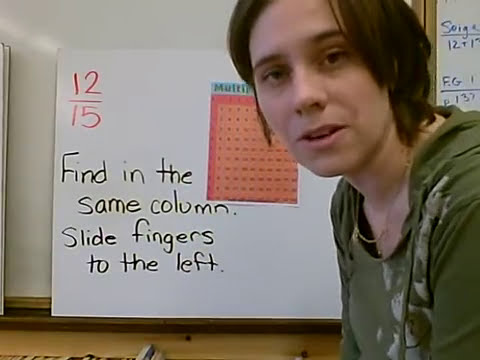This is an image of a young woman in her early to mid-20s, possibly a teacher or a student teacher, situated in a classroom setting. She has dark brown hair that is parted on the left, brushed over her forehead to the left, and cropped just below her chin at neck level. Her fair skin and dark eyebrows show she has no makeup. She is wearing an olive green hoodie over a green, rounded neck shirt, complemented by gold necklaces. 

The woman is positioned on the right side of the photograph. The top of her head and the right side of her body are partially cut off by the frame. She leans slightly into the picture, looking directly at the camera. 

Behind her, there is a whiteboard supported by a brown wooden ledge, with an array of educational materials displayed. A square white poster board prominently features the fraction 12/15 in red text at the top left corner. Below this, in black text, are the instructions: "find in the same column. slide fingers to the left." Adjacent to this text is a red grid that appears to be part of a multiplication table, with a light blue border at the top. The grid is partially obscured by the woman’s head. The overall scene suggests an educational environment, possibly involving math instruction.